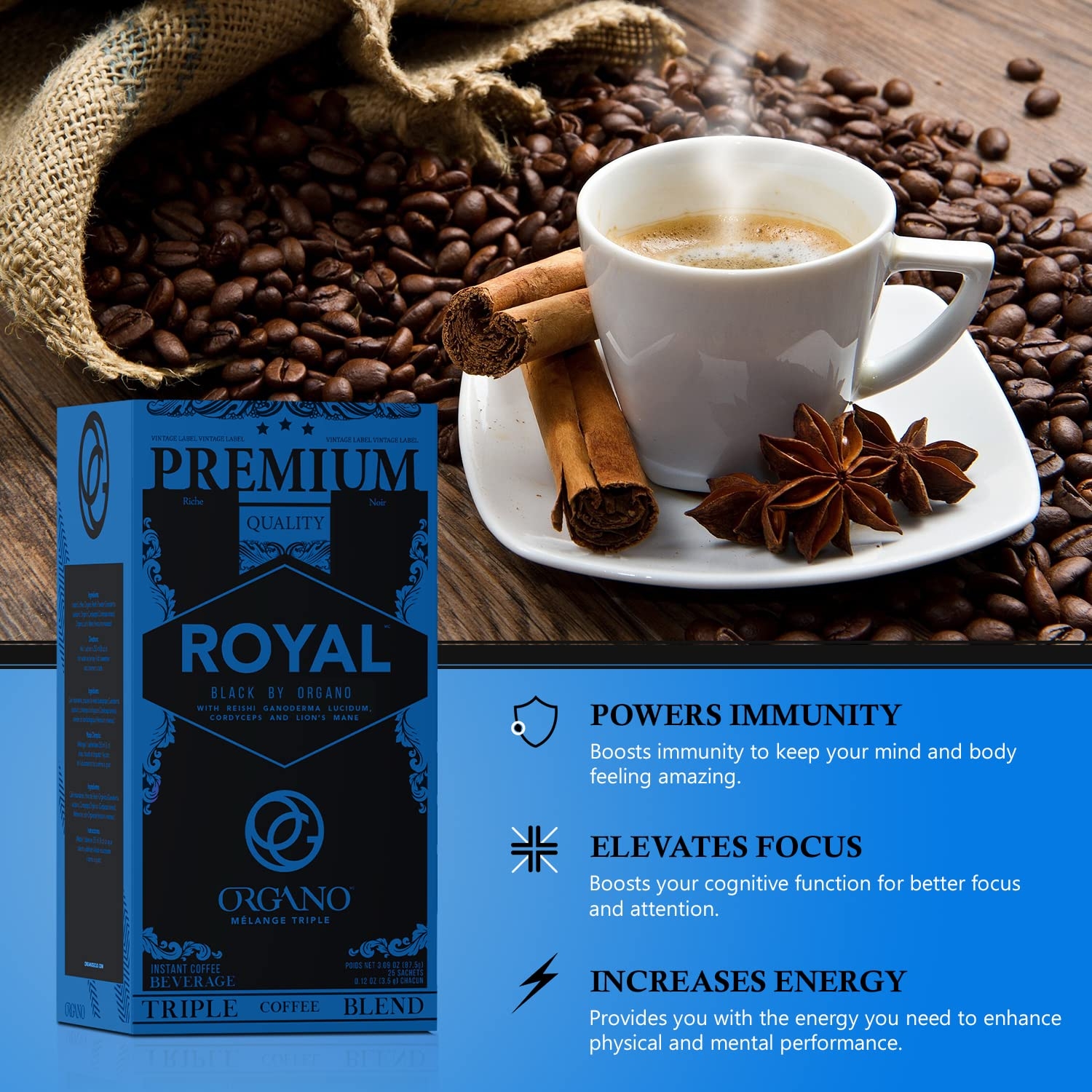The image showcases a detailed advertisement for a premium coffee blend called "Royal Black by Organo." At the center of the scene, a small white coffee cup with an arched handle sits on a matching white saucer. The cup is filled with brown coffee, topped with a bit of froth. Beside the cup, two cinnamon sticks and cinnamon clover or leaf decorations enhance the aesthetic appeal. 

This setup is placed on a wooden table, surrounded by an inviting spill of coffee beans that seem to have escaped from a tan burlap sack visible in the top left corner of the image. Above the cup, there's a small blue box resembling a cigarette pack, which carries the label "Royal Black by Organo Premium Quality Triple Coffee Blend." The blue box features texts in black and white, highlighting the product's benefits: "Powers Immunity," "Elevates Focus," and "Increases Energy" with corresponding symbols like a shield, a cross, and a lightning bolt for visual emphasis. The background and overall composition create a rustic and appealing advertisement, enhancing the premium feel of the coffee product.